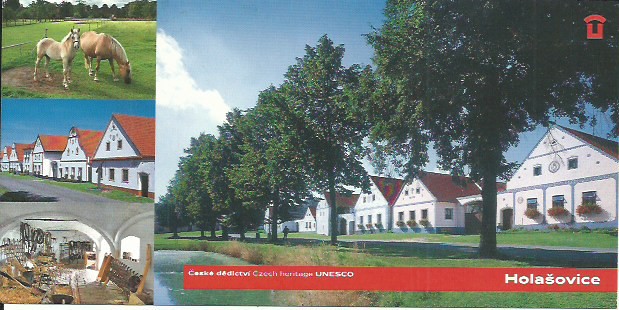The photograph depicts a beautifully landscaped farm scene, likely part of a UNESCO heritage site in the Czech region, possibly Holosovice or a similarly named place. The right side of the image features a row of white buildings, resembling barns or stables, distinguished by their reddish or brownish rooftops. These buildings are fronted by a path and a row of trees with green leaves and brown trunks. In the middle ground, several buildings and barns are visible, surrounded by manicured greenery. The foreground includes a group of beige horses grazing on the green grass. The bright blue sky arches over this peaceful countryside setting. On the bottom of the image, a red horizontal line with white text prominently displays "UNESCO" and "Holosovice." The left side of the photograph showcases a collage of three smaller images: the first focuses on the horses, the second shows a more detailed exterior view of the stables, and the third captures the inside of a barn, complete with horse tack, bridles, straw, and wheelbarrows.